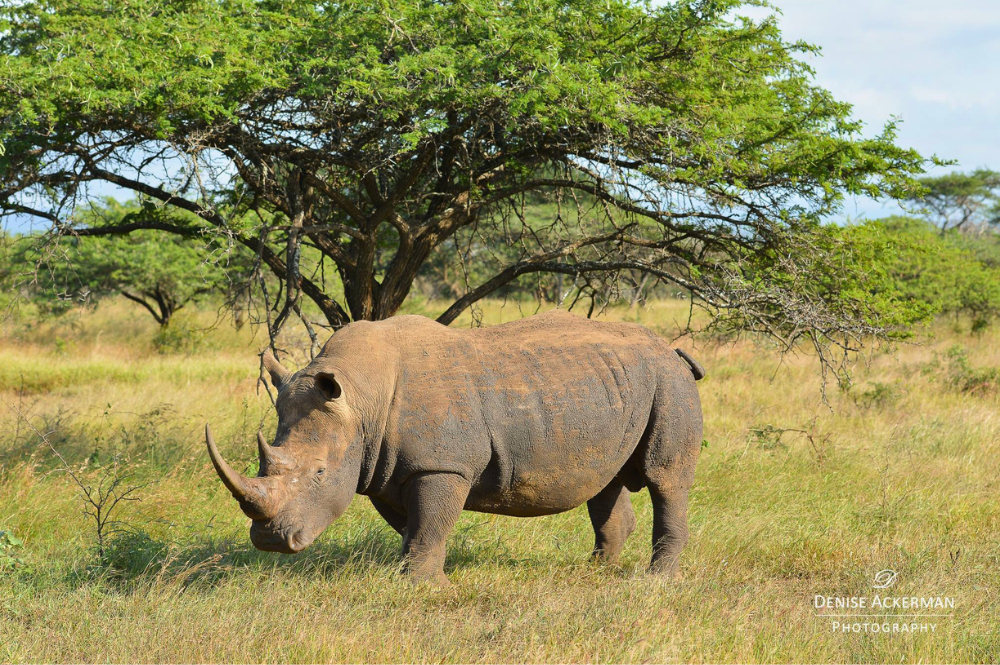This image captures a majestic rhinoceros, standing prominently at the center of the frame in an African savannah. The rhino, covered in a layer of dirt, has a dark gray, almost tan coloration, and is facing slightly to the left, showcasing its two impressive horns. Surrounding the rhino is a mix of green and slightly brownish grass, suggesting a season of transition. The background features several smaller, umbrella-shaped trees with dense green canopies and sprawling branches, providing scattered shade on the grassy landscape. High above, the sky is a clear blue with wispy white clouds stretching across the horizon. At the bottom right corner of the photo, "Denise Ackerman Photography" is elegantly written in white, marking the artist's work.